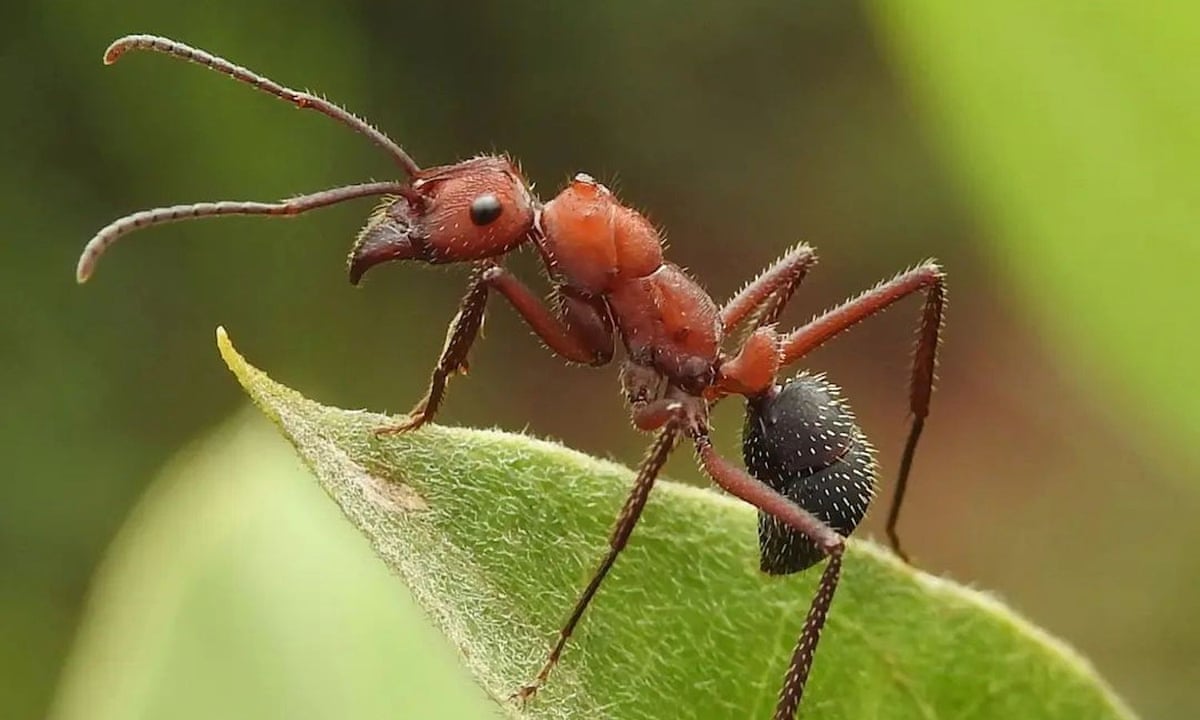The photograph is an extremely close-up, macro-style image taken outdoors during the daytime. The image, approximately 5 inches wide by 4 inches high, features a red ant standing on a green leaf covered in fine white hair-like fuzz. The ant, positioned with its head towards the left, showcases its two long, segmented antennae, each about an inch and a half long. The ant's head is red with black, protruding eyes and visible white hairs. One of its mandibles can be clearly seen near its mouth, which has a downward turn.

The ant's body exhibits a reddish-brown color with an amber undertone, transitioning to a darker hue towards its legs and culminating in a black posterior segment. The insect's six legs are notably long, with darker coloration towards the lower halves. The entire body is sprinkled with tiny white bristles. The background of the photograph is artfully blurred, displaying a mix of green and brown tones with a hint of yellowish light in the upper right corner, enhancing the depth of field and bringing the minute details of the ant and leaf into sharp focus.